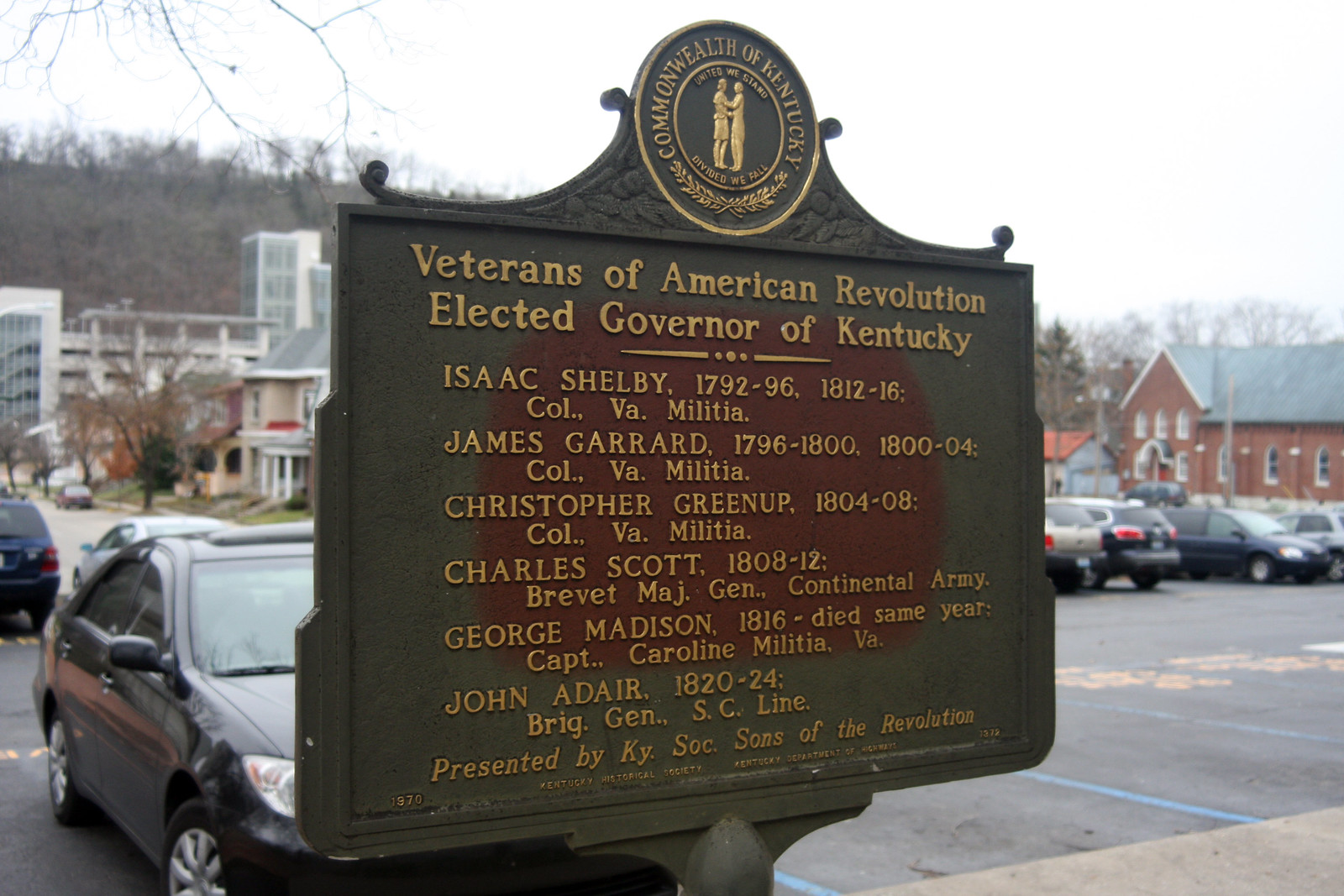The image depicts a rectangular, bronze-colored historical sign situated outdoors near a parking lot, with a backdrop of parked cars, various buildings, including a church and some houses. The sign, a memorial, features the seal of the Commonwealth of Kentucky at the top, adorned with a gold carving of two individuals shaking hands, framed by laurel leaves, and bearing the motto, "United We Stand, Divided We Fall." Below this emblem, the sign honors notable veterans of the American Revolution who were elected as governors of Kentucky. It lists Isaac Shelby, 1792-96 and 1812-16, Colonel of the Virginia Militia; James Garrard, 1796-1800 and 1800-04, Colonel of the Virginia Militia; Christopher Greenup, 1804-08, Colonel of the Virginia Militia; Charles Scott, 1808-12, Brevet Major General in the Continental Army; George Madison, 1816, Captain in the Caroline Militia, Virginia; and John Adair, 1820-24, Brigadier General of the South Carolina Line. The memorial was presented by the Kentucky Society, Sons of the Revolution.